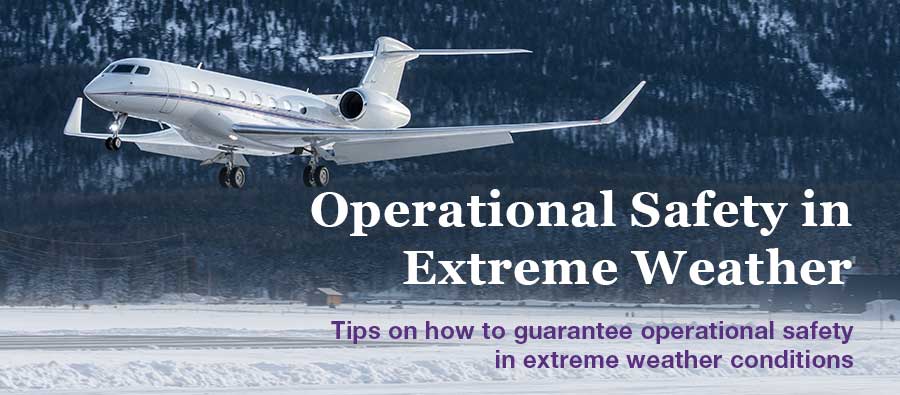The image is a rectangular frame, oriented such that its long sides stretch horizontally. Dominating the scene is a small white jet captured mid-landing, descending towards the left. The aircraft's landing gear is deployed, while its single rear-mounted engine and fully extended wings are clearly visible. Positioned slightly to the right within the frame, the jet stands out prominently against its snowy backdrop.

Across the upper portion of the image, bold white text reads, "Operational Safety in Extreme Weather." Directly beneath this, in smaller purple writing, the text continues with, "Tips on How to Guarantee Operational Safety in Extreme Weather Conditions."

The background is a stark white runway, blanketed in snow, enhancing the sense of a challenging winter environment. Two small structures are situated approximately a quarter of the way up from the bottom of the image. Further back, a dense, snow-covered wooded forest rises towards a gently sloping hill, adding depth to the wintry landscape.